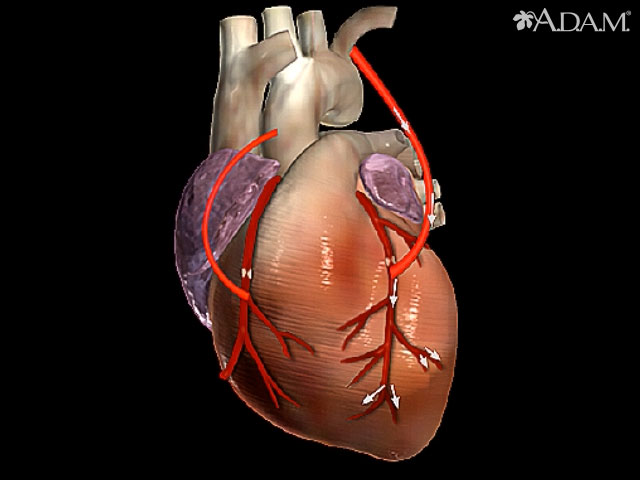This image is an artist's digital conception of a human heart set against a stark black background. Dominating the upper right corner is an emblem featuring the word "A-D-A-M" in white, each letter separated by periods, and a leaf attached to the letter "A." The heart itself is depicted in various hues, primarily reds, oranges, and occasional purples, giving it a vivid, synthetic appearance. Arrows, rendered in white, illustrate the flow of blood through the heart's major vessels, detailing the pathways through the aortas, ventricles, and atriums. Despite its diagrammatic elements, the image lacks any textual annotations explaining the specific parts of the heart. The overall composition suggests a blend of artistic interpretation and computerized design, possibly for educational or promotional purposes.